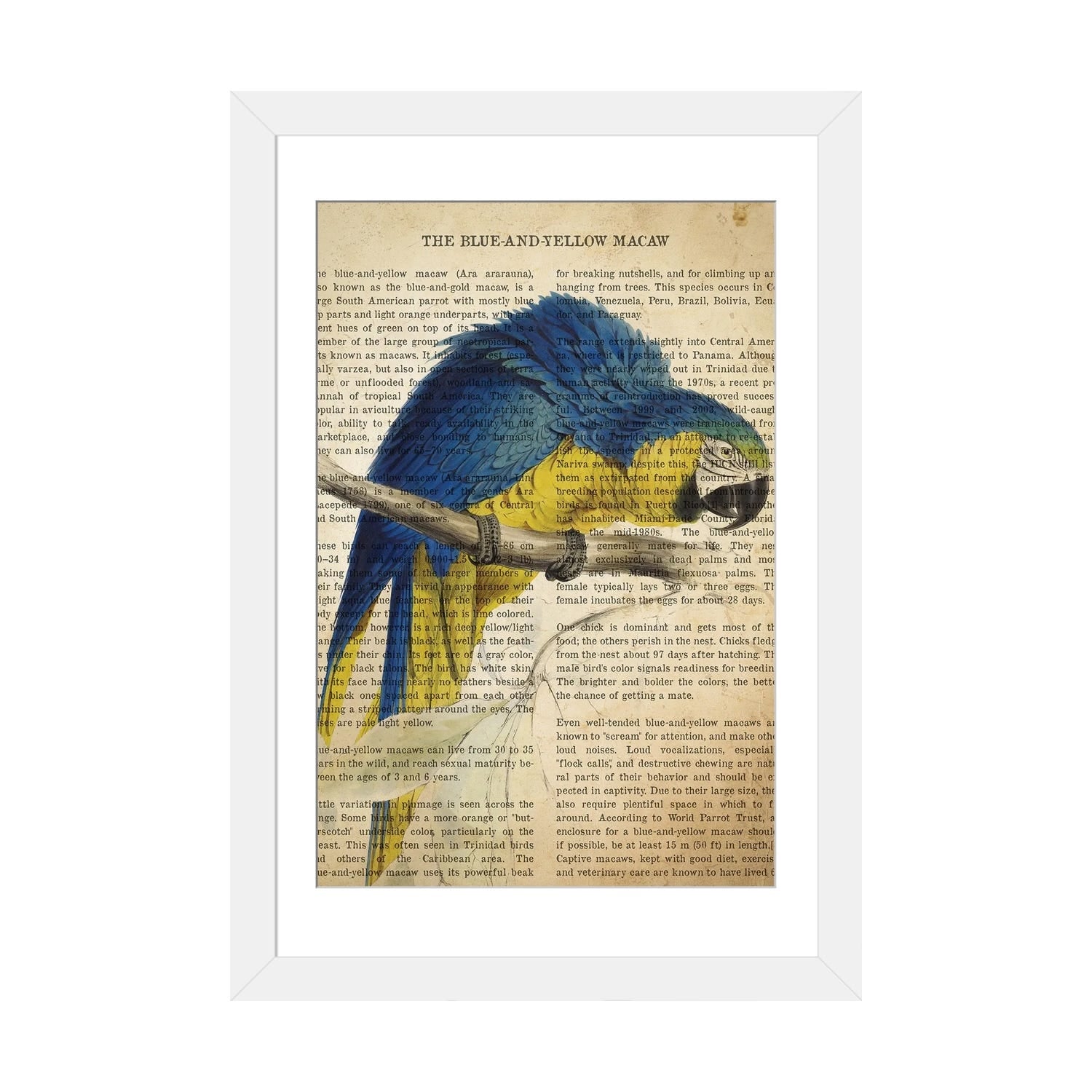The image depicts a vivid and intricately detailed illustration of a blue and yellow macaw, prominently titled "The Blue and Yellow Macaw" at the top. The illustration is set against an aged-looking piece of paper that gives the impression of an antique nature textbook or magazine page, with typewriter-style black font text forming two columns of descriptive paragraphs. The macaw, poised with its claws gripping a grey branch, displays its vibrant blue plumage on the back and yellow feathers on its chest, with a hint of white around its eye and a distinctive black beak. Uniquely, the bird appears semi-transparent, allowing the typed text to be visible through its colorful feathers. The macaw's head tilts towards the middle right of the page, while its tail extends toward the bottom left. The entire composition is framed by a white border, further enclosed by a light blue outer border, enhancing the vintage and illustrative quality of the image.